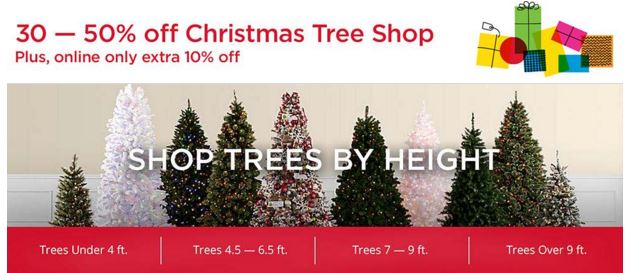This detailed description outlines the various elements present in a screenshot of a Christmas sale advertisement.


The top of the screenshot features a white horizontal banner with a white background and bold red text. In the top left corner, it prominently states "30-50% Off Christmas Treetop" in bold letters. Beneath this in smaller red font, it mentions "Plus, Online Only Extra 10% Off." 

The right side of the banner showcases stylized, semi-transparent, overlapping images of modern-looking gift boxes arranged symmetrically. These gifts come in various colors – yellow, green (vertical), blue, pink – giving a vibrant, festive feel.

The center section of the image highlights a collection of Christmas trees of varying sizes and types, arranged somewhat symmetrically. Most trees are green, except for a notable white tree at the center adorned with red and green decorations. Flanking this centerpiece, additional white trees appear, adding to the symmetrical balance. Some trees are tall, while others are short.

At the bottom is a red horizontal banner with white text, categorizing the trees by size: "Trees Under 4 Foot," "Trees 4.5 to 6.5 Feet," "Trees 7 to 9 Foot," and "Trees Over 9 Foot." This section helps customers easily navigate their options based on tree height.